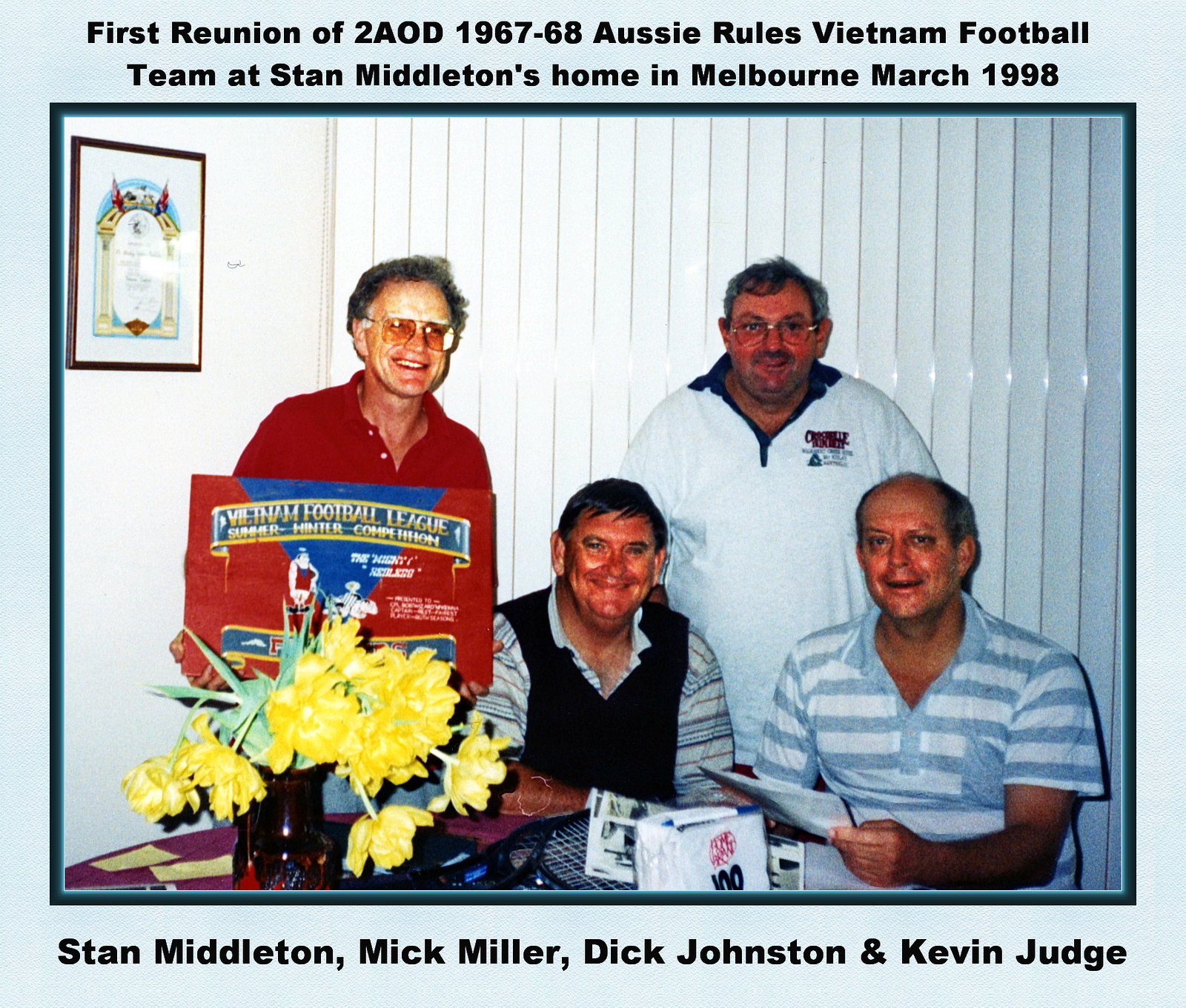This photograph captures a joyous reunion of the 2AOD 1967-68 Aussie Rules Vietnam Football Team held at Stan Middleton's home in Melbourne, March 1998. Four older gentlemen, identified as Stan Middleton, Mick Miller, Dick Johnston, and Kevin Judge, are the focal point of the image. The men, likely in their 60s or 70s, are all wearing casual polo shirts and sporting bright smiles, showcasing their camaraderie. The setting appears to be a dining room with vertical Venetian blinds behind them, indicative of a homey atmosphere. Two of the men are seated at a table adorned with a vase of yellow flowers, a napkin holder, and what appear to be parts of tennis rackets. Behind the seated men, the other two team members stand, alluding to a historical connection as one of them holds a sign that reads "Vietnam Football League Summer Winter Competition." The background includes a plaque and framed items on the wall, part of which appears to display text, adding to the memorabilia of the occasion. The borders of the photograph feature text in a light blue frame, with a prominent banner in red and blue stating "Vietnam Football League."